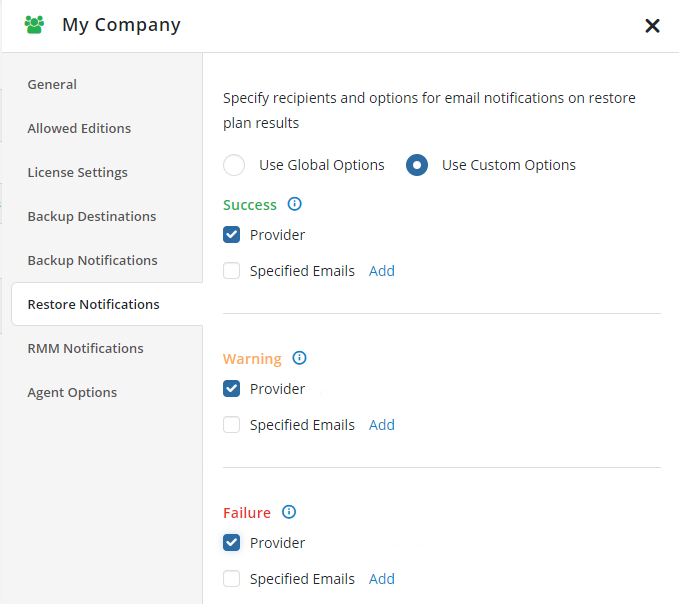The image depicts a detailed user interface for a software management system under the header "My Company," displayed in a dark gray font at the upper left corner, next to three green silhouettes of users. The interface transitions into a light gray background with medium gray text listing various menu options.

The menu options are: 
- General
- Allowed Editions
- License Settings
- Backup Destinations
- Backup Notifications
- Restore Notifications (highlighted in white with a light gray border)
- RMM Notifications
- Agent Options

On selecting "Restore Notifications," a panel appears on the right with the header in black text: "Specify Recipients and Options for Email Notifications on Restore Plan Results." 

Within this panel, there are two circular tick boxes:
1. "Use Global Options" (not selected)
2. "Use Custom Options" (selected)

Following this, "Success" is highlighted in green, accompanied by an info bubble to its right. Below it, the options "Provider" and "Specified Emails" are present with square checkboxes next to them. The "Provider" option is selected, filled with a dark navy blue and displaying a white checkmark. To the right of "Specified Emails," there is a blue "Add" option.

A gray line serves as a divider, followed by "Warning" highlighted in orange with an adjacent info bubble. Similar options ("Provider" and "Specified Emails") are listed, with the "Provider" option selected. The "Add" button appears to the right of "Specified Emails."

Another gray divider line follows, leading to "Failure" marked in red, accompanied again by an info button. The "Provider" option in this section is selected, while "Specified Emails" is not.

The layout clearly organizes options and settings for managing restore notifications, with a consistent use of color and icons to denote different states and actions.